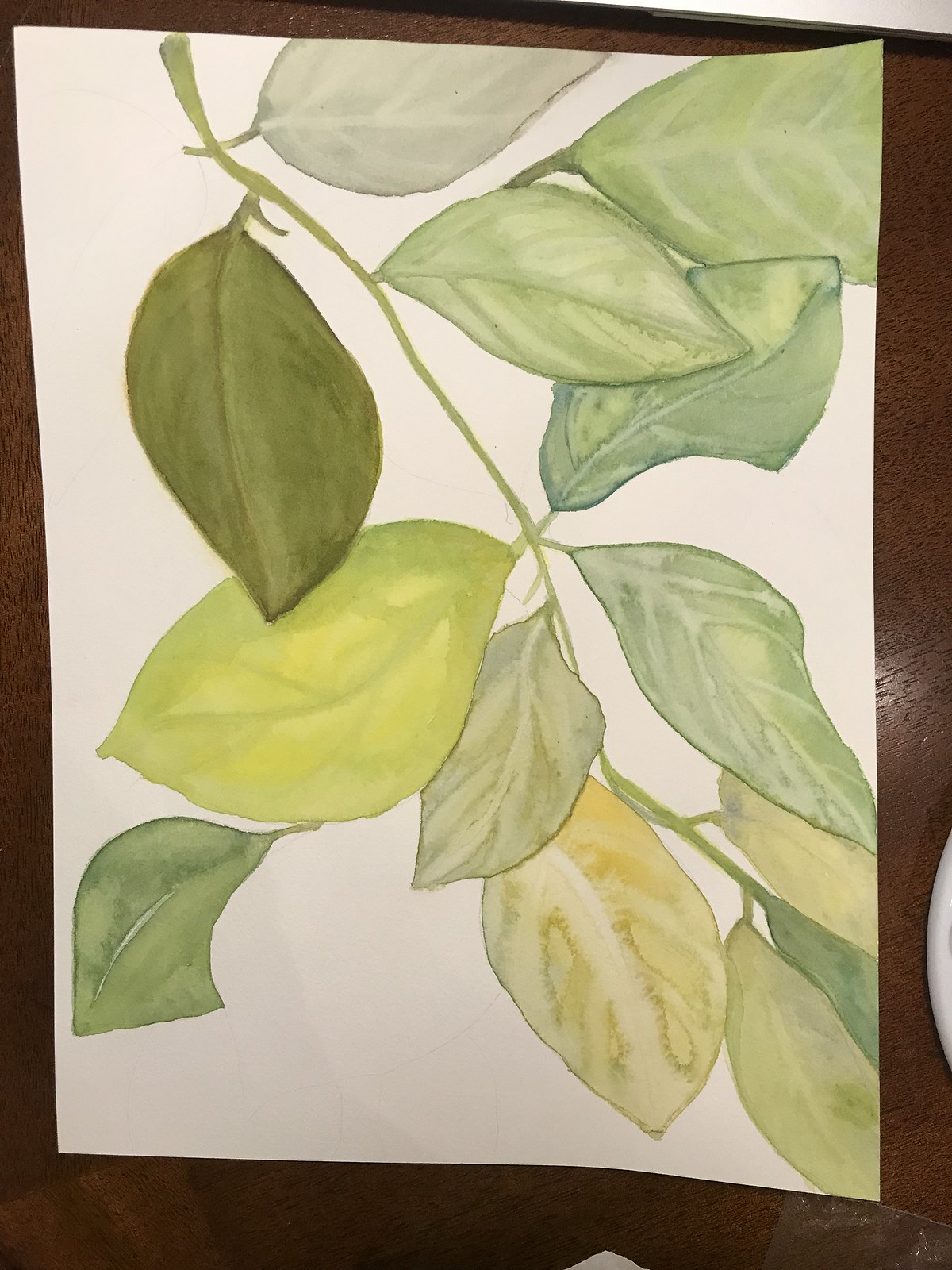In this image, a white, square piece of paper is placed on a dark brown table. The paper features a detailed sketch of various leaves all connected by a single vine, which begins at the top left corner and trails downwards. The first leaf on the right side of the vine is colored gray, while the other leaves exhibit shades of green. Some of the leaves, particularly at the bottom, have yellow hues or are a mix of yellow and green. The bottom right corner of the image shows part of a plastic cover, and there is a curved white object partially visible on the right side. The table's dark brown surface is seen along the bottom, right, left, and top edges of the image, framing the sketch.